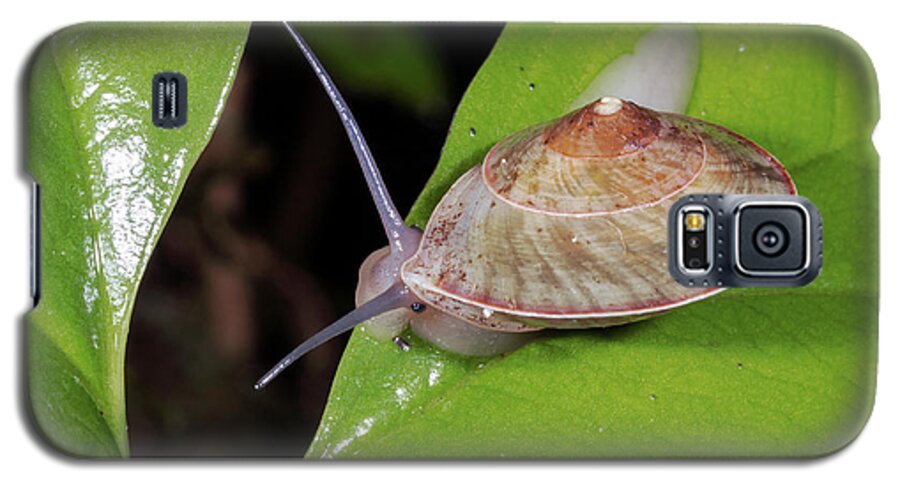The image is of the back of a phone case that features precise cutouts for the camera, microphone jack, and charging port. The phone case is primarily designed with nature-inspired graphics. The left side of the case shows a small portion of a green leaf, while the right side features a larger, detailed green leaf. Perched on the right leaf is a snail with a reddish-brown, spiraled shell adorned with hints of green, tan, and white. The snail's body is a translucent mix of purplish and whitish hues, and it has two long antennas extending beyond the edge of the leaf. The snail's eyes are noticeable, and it appears to be nibbling on the leaf's edge, creating a realistic and vivid depiction of a natural scene.